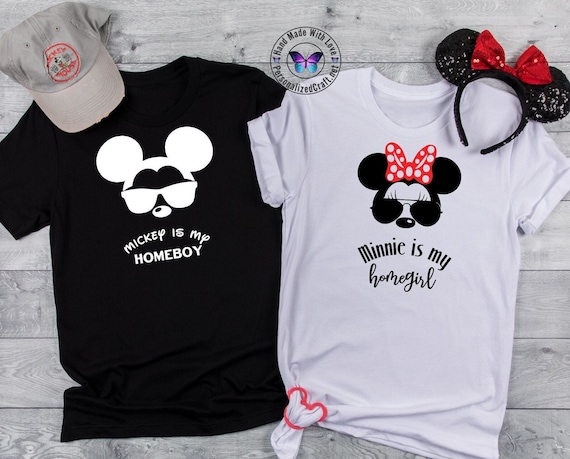This image features an overhead shot showcasing a pair of stylish t-shirts and accompanying accessories, ideal for fans of Disney. On the left, a black t-shirt sports a white silhouette of Mickey Mouse’s ears and nose, complete with sunglasses, and the phrase "Mickey is my homeboy" written in bold white letters. To the right, a white t-shirt features a similar design with Minnie Mouse's ears, and she dons sunglasses and her iconic red bow with white polka dots. This shirt is emblazoned with "Minnie is my homegirl" in black letters.

Adjacent to the white t-shirt, a Minnie Mouse headband with red ears and a bow is positioned, enhancing the whimsical theme. In addition, a gray hat lies near the black t-shirt, adorned with a red circular decal that includes a full-body image of Mickey Mouse in his red pants and the words "Mickey" above and "Mouse" below in red lettering.

Both t-shirts are tastefully arranged on a gray wooden surface, adding a rustic charm to the presentation. At the top center of the image, there is a circular logo that reads "handmade with love" and "personalizedcraft.net" both at the top and bottom of the circle, featuring a colorful butterfly with purple upper wings and teal lower wings.

Adding a unique touch, the white t-shirt incorporates a scrunchie styled to resemble Mickey or Minnie's head, making it as functional as it is fashionable. This detailed and thoughtfully curated scene exudes a handcrafted appeal, perfect for an Etsy product listing.